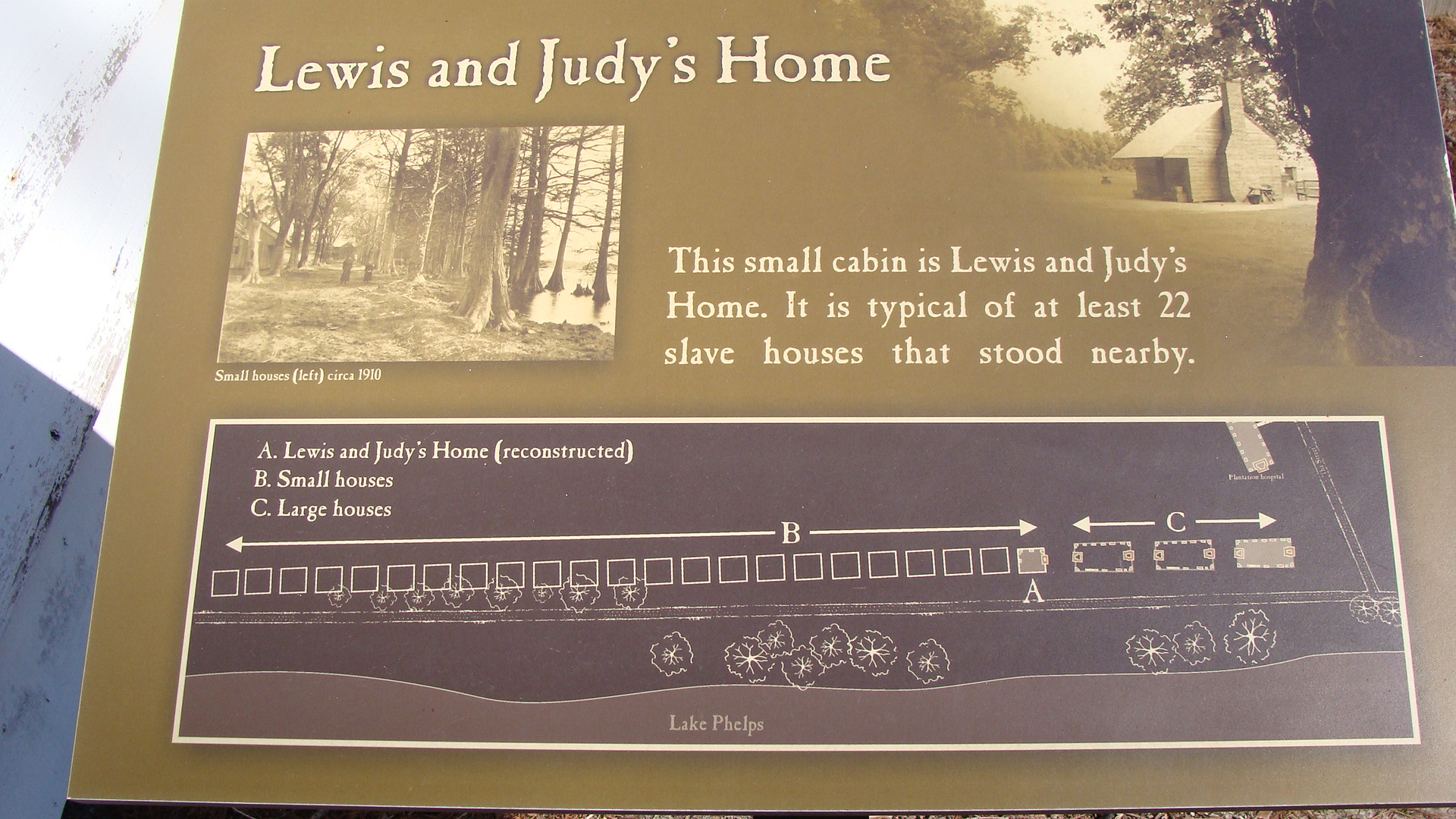The image features a detailed brown sign titled "Lewis and Judith's Home." Highlighting historical context, the sign mentions that the small cabin depicted is typical of at least 22 slave houses that stood nearby. To the left of the sign is an illustration showing a dense forest with many tall trees and two people walking among them. On the right side, there's an image of the actual cabin positioned next to a large tree, with a backdrop of sky and woods. Below, a detailed diagram maps out the area, labeling "A. Lewis and Judith's Home Reconstructed," "B. Small Houses," and "C. Large Houses," complete with arrows for guidance. The sign’s palette includes black, white, green, olive, off-white, dark brown, light brown, and sepia tones, providing a neutral yet informative visual experience.